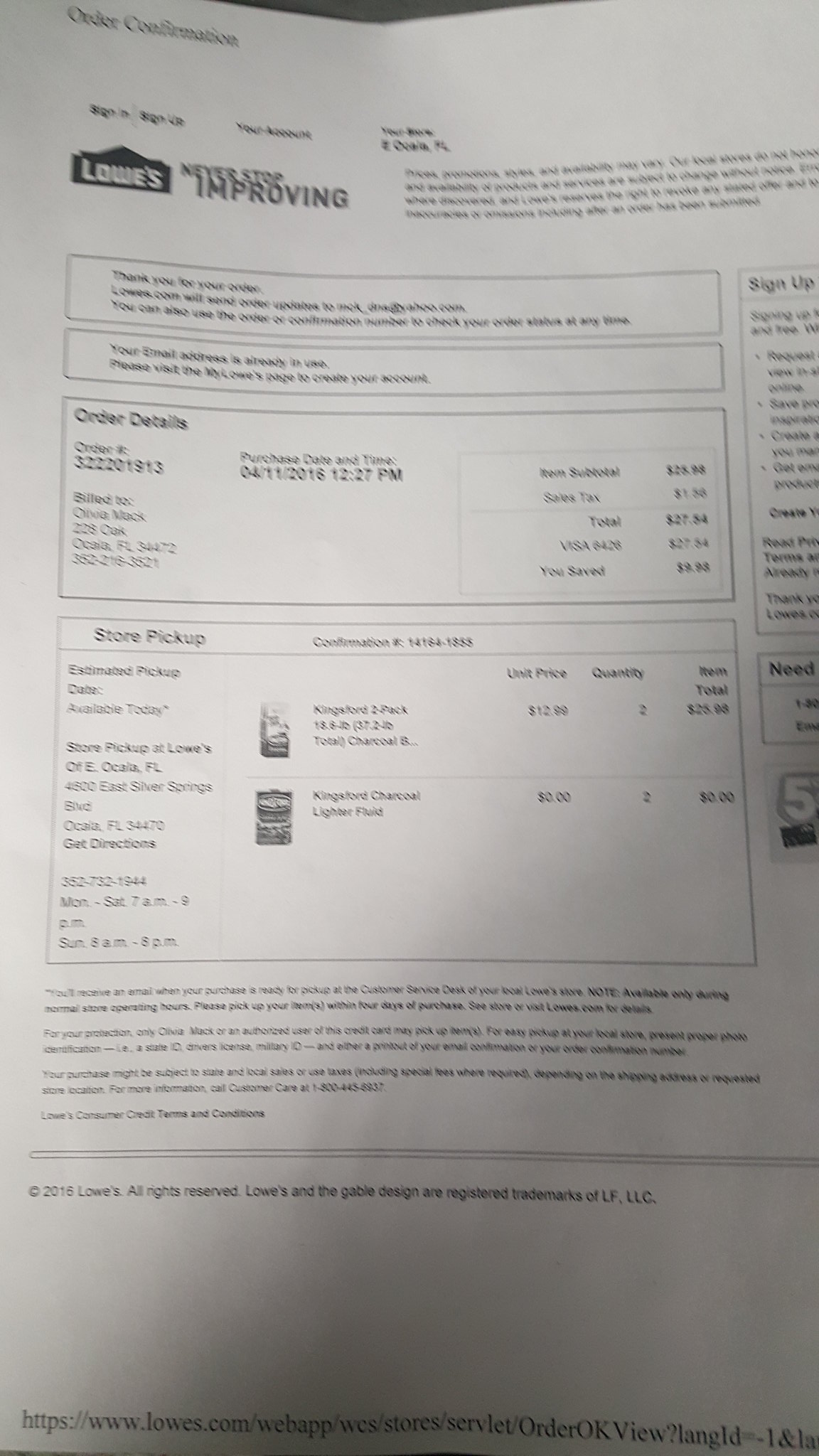This image displays an order confirmation receipt from Lowe's. At the top, the document features the classic Lowe's logo accompanied by their slogan, "Never Stop Improving." Below this, there's a disclaimer and various confirmation details originating from the website, indicated by the URL "Lowe's.com" at the bottom.

The receipt is addressed to someone named Olivia, who resides in Florida. It includes a timestamp indicating the purchase was made in the afternoon of April 2016. The order totals around $27, including sales tax, and it notes the savings achieved on the purchase.

Detailed order information reveals that Olivia placed a pickup order for charcoal and lighter fluid, suggesting plans for a barbecue. Interestingly, the lighter fluid was included at no cost. Additional terms and conditions, copyright information, and partial instructions for setting up an online account are visible. However, some of the text on the right side is cut off, showing only fragments like "sign up," "need," and a toll-free number.

In essence, this image is a detailed and itemized order confirmation from Lowe's, providing comprehensive information about Olivia's purchase and instructions for collection.